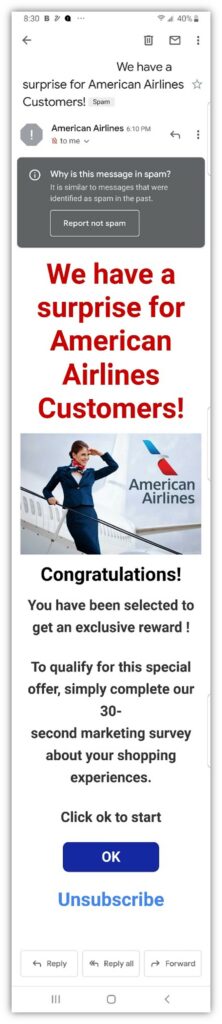**Email Screenshot with Potential Spam Alert from American Airlines**

The image appears to be a poorly-rendered screenshot of a mobile device's screen, specifically showing an email marked as spam. The overall quality of the screenshot is low, and the image seems stretched.

### Email Details:
- **Sender:** American Airlines
- **Subject:** "We have a surprise for American Airlines customers" (highlighted in bright red font)
- **Spam Notification:** 
  - The email is marked as spam, indicated by a gray box featuring an eye icon and a message: "Why is this message in spam? It is similar to messages that were identified as spam in the past."
  - Below the notification, there is a button labeled "Report not spam."

### Email Content:
1. **Header Image:**
   - The email includes an image of a female flight attendant in a smart blue uniform, complete with a red and blue neck scarf.
   - The flight attendant is facing forward with an airplane and the American Airlines logo in the background.

2. **Main Offer:**
   - Below the image, the text reads: "Congratulations! You have been selected to get an exclusive reward."
   - To qualify for the reward, recipients are instructed to "complete a 30-second marketing survey about your shopping experience."
   - Beneath this instruction, a blue button with the label "OK" invites users to begin the survey.

3. **Footer:**
   - At the bottom of the email, the word "unsubscribe" is displayed, presumably as a link to opt-out of future communications.

This apparent promotional email from American Airlines, marked as spam, invites recipients to participate in a survey for a special reward. The image quality and potential phishing elements warrant caution.